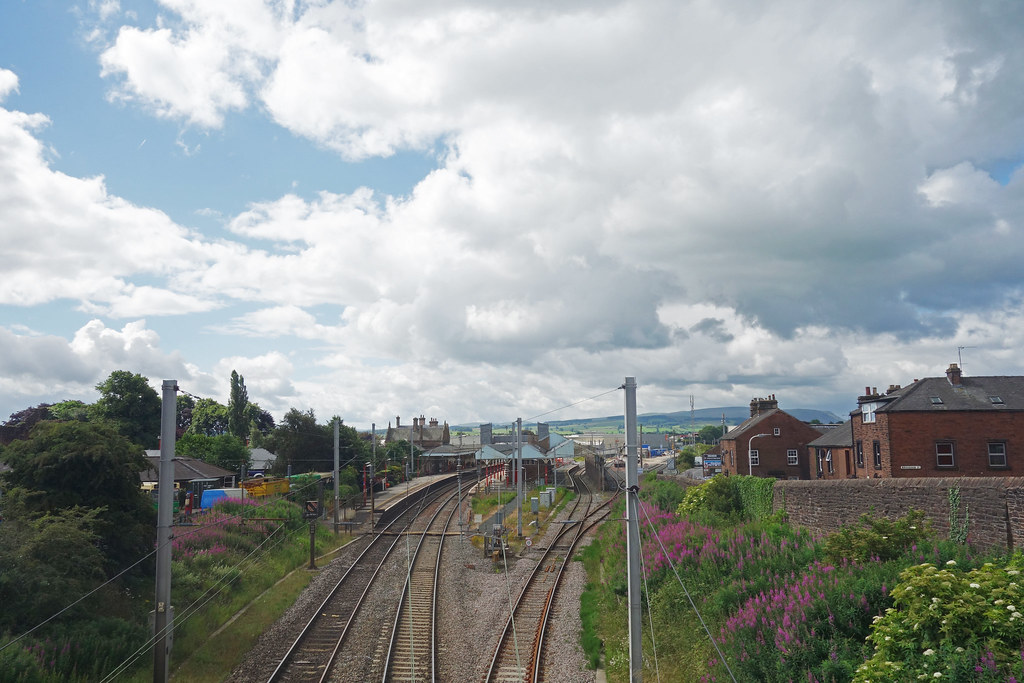This elevated photograph captures a detailed, expansive view of a small town's railroad system amidst a cloudy sky. In the foreground, three railroad tracks run across the image, with two situated towards the left and one towards the right. These tracks evolve into multiple paths, with the rightmost track splitting into two further down. The landscape alongside the tracks is rich with green plants and shrubbery, including lavender and white-flowered bushes. To the right, three large, two-story brick buildings with dark gray roofs and black window panes sit behind a tall brick wall, partially obscured by the plants in front. The left side of the image features a combination of homes, additional shrubbery, and trees. In the distance, beyond the train tracks that lead towards a gray-roofed train station, various service buildings are visible. The backdrop is marked by cloudy skies with a hint of blue, and faint mountains can be seen in the background, adding depth to the scene.